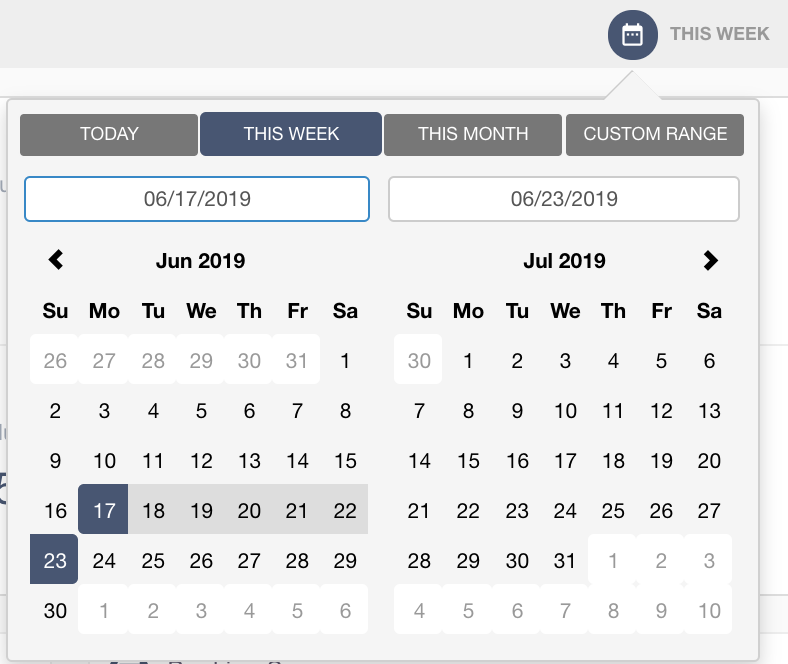The image features a calendar interface prominently displaying two months: June 2019 on the left and July 2019 on the right. Positioned on the top right corner, there is a label stating "This Week" accompanied by a calendar icon. Above the calendar, there are navigation tabs labeled "Today," "This Week," "This Month," and "Custom Range." These tabs are written in white and have a grey background, except for "This Week," which is highlighted in blue, indicating it is currently selected.

On the left side, immediately below "This Week," the date range 6-17-2019 to 6-23-2019 is outlined in blue. Within the June 2019 section, dates from the previous month of May are displayed in grey with a white background. The current dates for June are displayed normally, with June 17 (a Monday) and June 23 (a Sunday) highlighted in blue, indicating the selected week. The days in between these highlighted dates are marked in grey.

In the July 2019 section on the right, the remaining days for the upcoming month are also presented with a white background. The overall calendar background is white. This detailed structure offers a clear visual representation of the selected week and differentiates between the days of the current and adjacent months.